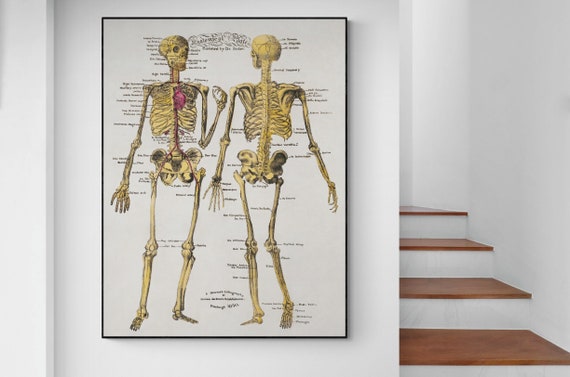The image is a horizontal-rectangular photograph of the interior of a home, featuring a white wall with a framed poster on the left and a staircase on the right. The poster, framed with a thin black border and set against a white background, depicts two yellowish-beige human skeletons—one viewed from the front and the other from the back. Each skeleton is heavily labeled with black text indicating various bones and anatomical structures. Notably, the heart is depicted in red, and blood vessels extend down through the leg bones. The staircase to the right has four wide steps with brown wooden tops and white risers, also surrounded by white walls. The right skeleton has its arms slightly moved, while the left skeleton has its arms positioned straight out. The overall shadow effect around the poster enhances the prominence of the skeleton images.